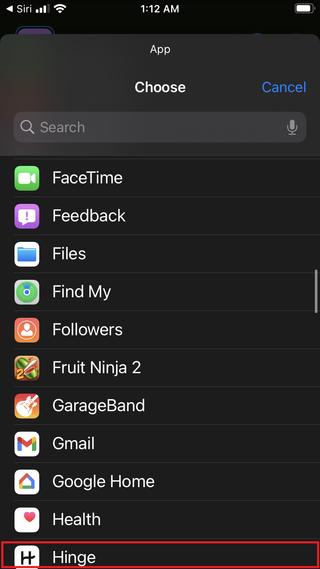This is a detailed screenshot of a phone's app list interface. At the top of the screen, elements of the phone’s UI are visible, including 'Siri' displayed in the top-left corner, signal bars, a Wi-Fi icon, the time '1:12 a.m.' centered, and a nearly full battery icon on the top-right corner. Below this section is a grey bar with 'App' on the left, 'Cancel' on the right, and a search bar situated underneath it, featuring a magnifying glass icon on the left and a microphone icon on the far right.

The main portion of the screen displays a list of apps against a black background. Each app entry consists of an icon on the left and the app's name on the right. The apps listed include FaceTime, Feedback, Files, Find My, and others, totaling eleven items. Notably, the last app on the list, named 'Hinge,' is highlighted with a red box around it, drawing attention to it among the other apps.